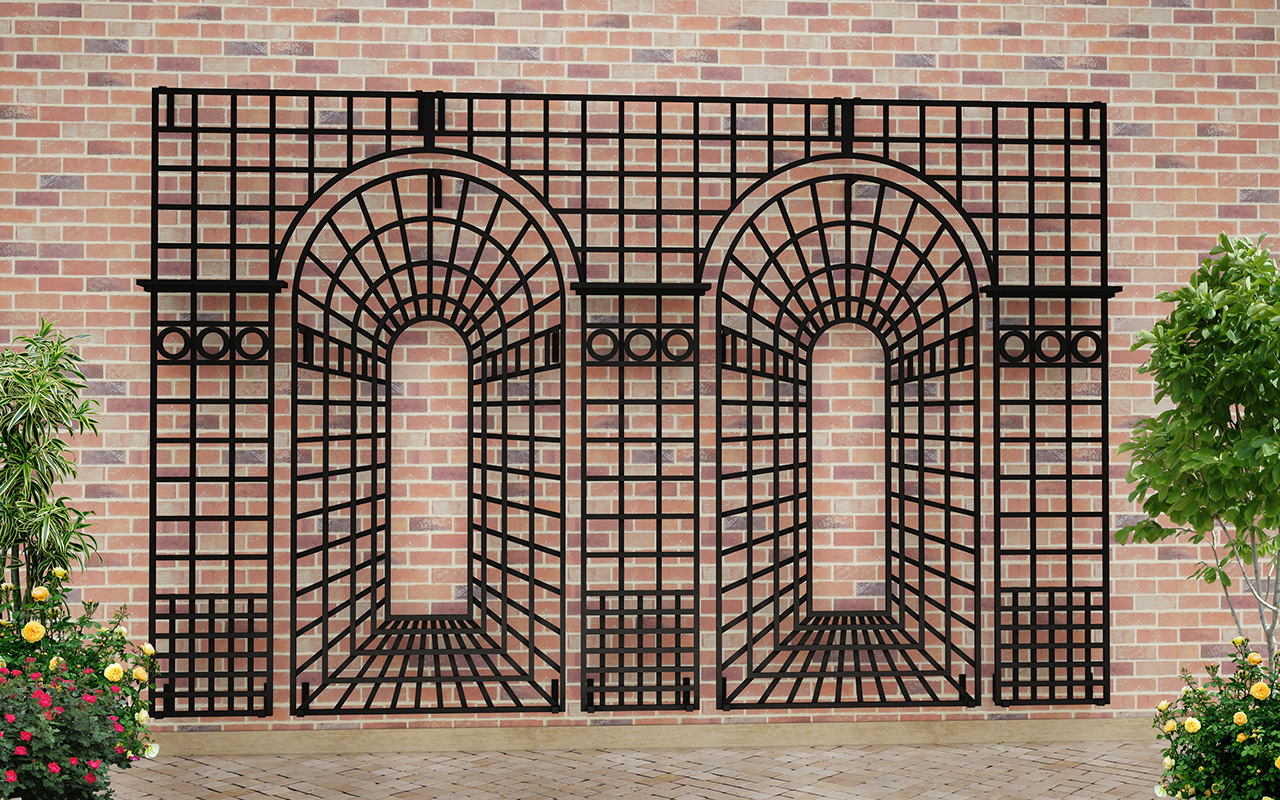This photograph, taken outdoors during the daytime, captures a large, ornate, black metal fence panel or trellis set against a multi-colored brick wall featuring shades of red, gray, and light orange. The trellis, designed to resemble two archways, gives off a three-dimensional effect, as if someone could walk through them, although it is actually a flat, single panel. The ground in front of the panel is covered with medium brown and gray brick tiling, enhancing the illusion of depth.

Framing the focal point of the black metal structure are vibrant bushes. To the left, you find a mix of green, yellow, and red flowers, with an abundance of small bright yellow and pink blooms that resemble a short shrub or possibly a lemon tree in appearance, though it is significantly shorter. To the right, a similar green bush with predominant yellow flowers is present, alongside branches that extend into a small green tree. The overall scene combines the elements of organic plant life and intricate man-made craftsmanship, creating a visually compelling outdoor art piece.